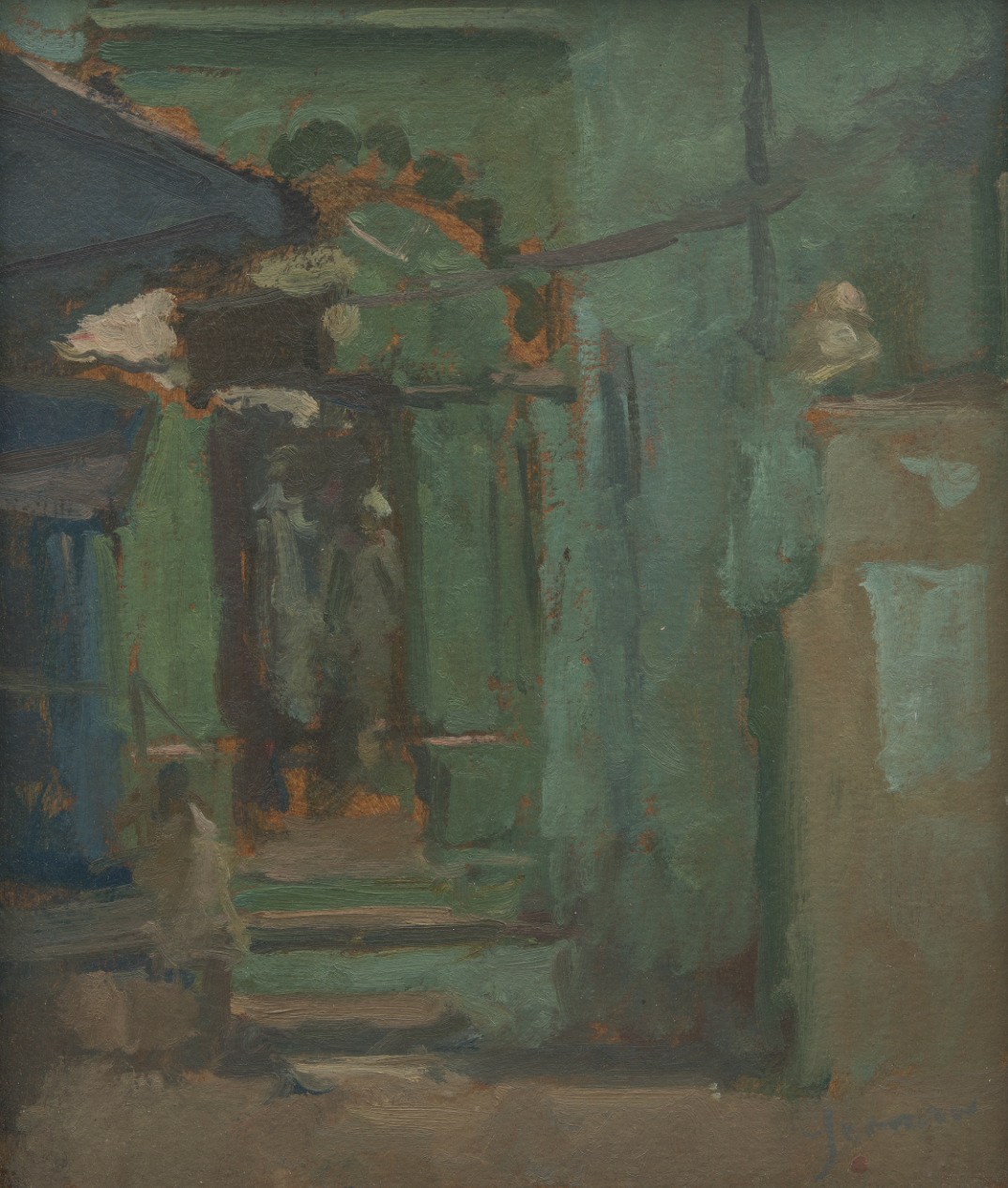This painting, executed in a modern, abstract style reminiscent of Picasso, features a blend of green, gray, and blue hues that create a blurred and indistinct scene. Dominating the composition is a green wall of a building with an arched doorway at its center. The doorway is framed by horizontal brown stripes that suggest steps, leading down to a brown, empty ground. To the left of the steps, there is a faint depiction of a blue building with hazy blue-green streaks. 

Amid the abstraction, you can discern several ghostly human figures. On the steps, there appears to be one person and potentially another smaller figure, indicated by a slightly triangular shape with dark and light brown accents. These figures seem to blend into the green background, contributing to the overall ambiguity. Within the doorway, there are two lighter, shadowy figures in grayish-blue tones, standing under the arch. 

The painting is characterized by a lack of clear boundaries, with elements bleeding into each other, creating a dreamlike, almost surreal visual experience. Set in portrait orientation, the artwork’s abstract nature invites multiple interpretations and a deeper engagement with its layered texture and forms.